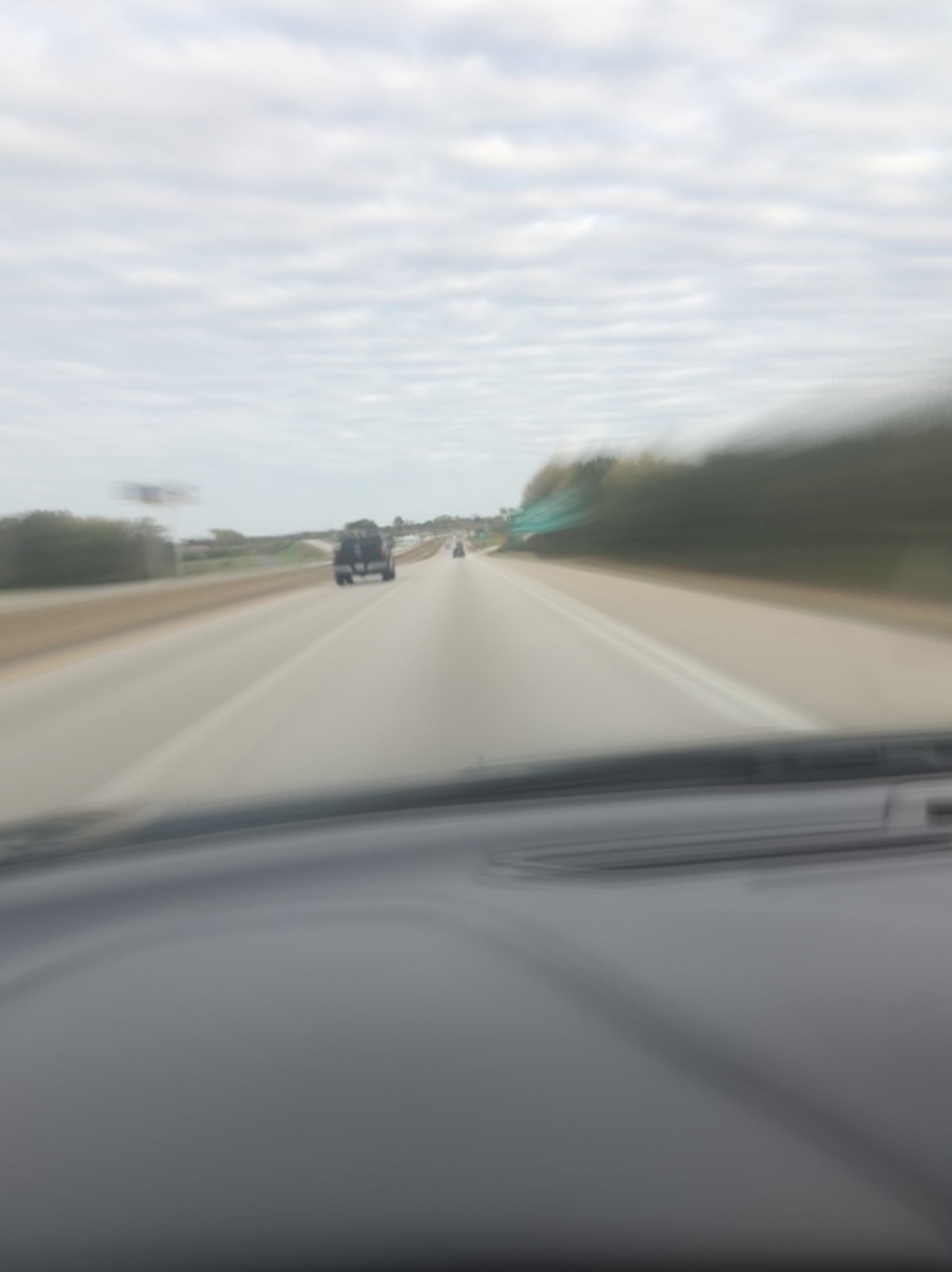The image captures the view from inside a moving vehicle on a highway. The camera angle, positioned from either the window or dashboard, offers a direct perspective of the road ahead. The concrete surface of the highway is marked with distinct white lines. In the distance, on the right-hand side, there is a blurry green highway sign. On the left side of the road, a black-colored truck is visible. The scenery is flanked by tall trees and abundant greenery, which appear blurred due to the vehicle's high speed. The vehicle’s dashboard is also in view, providing a sense of the interior space. Above, the sky is filled with thick, white, chunky clouds, completing the dynamic scene.